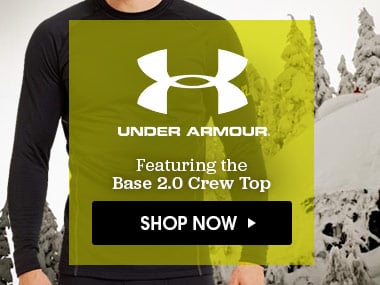This image captures a screenshot of a website showcasing an Under Armour product. The main background features a partially visible person, shown from the neck down, wearing a long-sleeve black shirt and black pants. The setting behind them includes a sky and a snow-covered hill adorned with snow-laden trees.

Prominently overlaid on the person's torso is a neon yellow square. Within this square is a white graphic resembling a large 'H', the recognizable logo for Under Armour. Accompanying the logo, the text "Under Armour" is prominently displayed.

Below this, the text "Featuring the Base 2.0 Crew Top" is indicated, highlighting the specific product being showcased. At the bottom of the image, a long black rectangular box features the text "Shop Now" in white. Adjacent to this text is a right-pointing triangle, signaling that this element is clickable, leading users to order the Under Armour product.